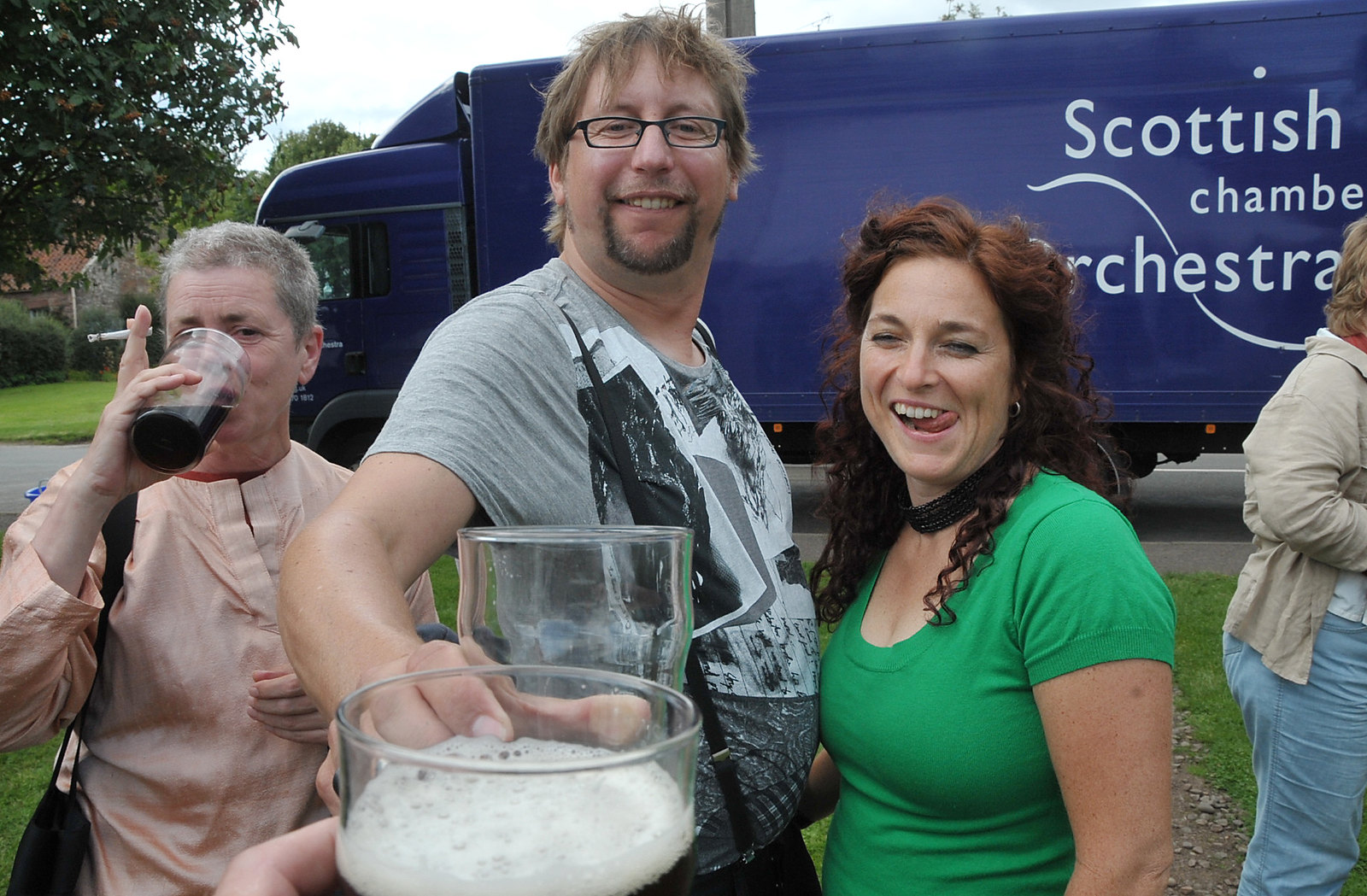In this vibrant outdoor festival scene, three individuals, all Caucasian, are evidently enjoying beers together in front of a large blue bus marked "Scottish Chamber Orchestra" in white letters. The celebratory moment captures a toast between the center man and the unseen photographer holding a foamy glass of dark beer. The central figure, a man with shaggy light brown hair, black-rimmed glasses, and a gray graphic tee, extends his glass forward with a grin. Flanking him on either side are two women. To his left stands a woman with short gray hair, dressed in a tan shirt, sipping from a glass of dark liquid while holding a cigarette and a purse over her shoulder. To his right, a younger woman in her 30s with curly reddish-brown hair dons a green T-shirt and playfully sticks her tongue out. The scene, set on a grassy lawn framed by a tree and a distant building, exudes a lively, communal atmosphere.